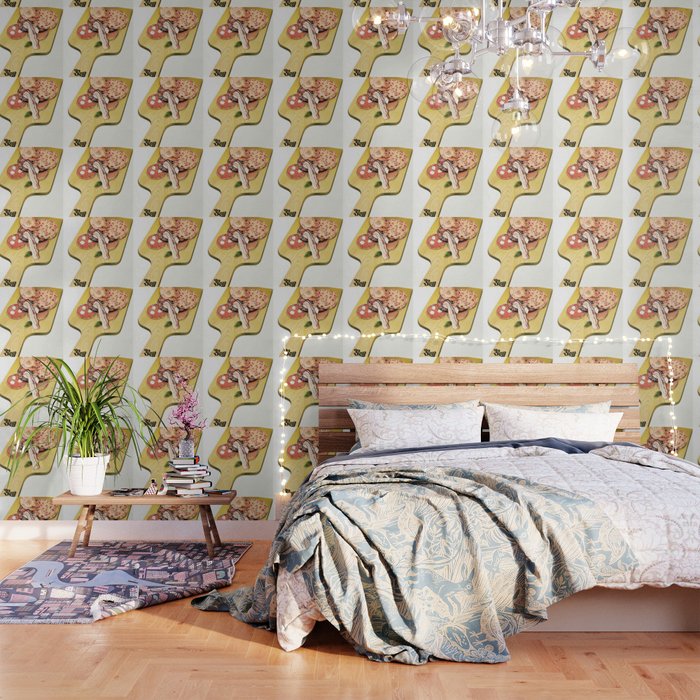This image is a detailed photograph of an indoor bedroom scene, captured in a square frame approximately six inches by six inches. The overall setting includes parquet light brown wood floors and a bed situated on the right-hand side of the image. The bed features horizontal wooden slats for the headboard, adorned with a string of white lights, and is covered with a light blue coverlet decorated with bird and bunny motifs. The bed also has a big white comforter with blue shading and is piled with four pillows.

To the left of the bed, a low wooden bedside table holds a large potted green plant, possibly a ficus, set in a white pot, and a stack of books topped with a small pink bonsai tree. Below this table lies a small rectangular rug, predominantly blue with pink rectangles.

Dominating the background is a unique off-white wallpaper adorned with a repeating pattern of wooden paddles holding assorted food items, likely pizza toppings or charcuterie, in squares with gray backgrounds. The chandelier, made of clear glass, hangs just right of the center at the top of the image, adding a subtle touch of elegance. The scene is accentuated by the intricate details of the wallpaper, the carefully arranged bedroom furniture, and the softly lit ambiance provided by the chandelier and string lights.